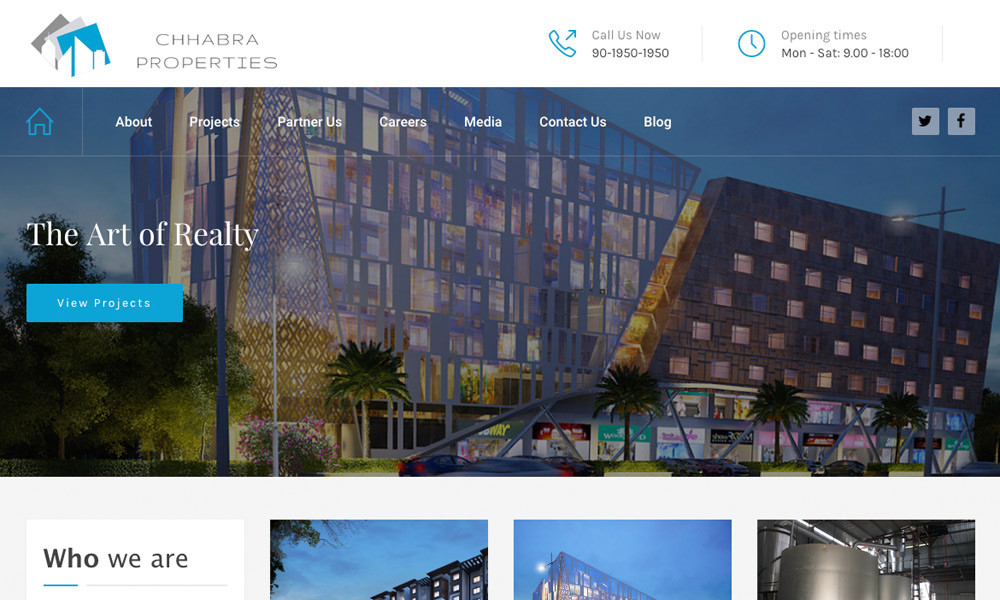This is a detailed screenshot of the Chabra Properties website, a real estate platform.

At the top of the website, there is a prominent white header. In the top-left corner, it features the Chabra Properties logo along with the company name "Chabra Properties" in a light gray, futuristic font. The top-right corner includes a blue phone icon beside the text "Call Us Now 9019501950" in gray. Adjacent to that, there's a blue clock icon indicating the opening times: "Monday through Saturday 9 to 18."

Below this header, there is a main image displaying one of their properties: a vibrant mall framed by palm trees. The front of the mall showcases a variety of stalls and a visible subway entrance.

The website's navigation menu is highlighted in a light blue banner, indicating that the "Home" section is currently active. Other clickable links include "About," "Projects," "Partner Us," "Careers," "Media," "Contact Us," and "Blog." Additionally, the top-right area of the screen provides clickable icons for Twitter and Facebook.

Superimposed on the main image is the tagline "The Art of Realty" in white text. There's also a light blue button labeled "View Projects" inviting users to explore more real estate offerings. Below this, a light gray section begins with the header "Who We Are," though the text is cut off and not fully visible. 

Alongside this section are three smaller images representing different Chabra Properties' real estate projects, partially cut off by the edge of the screenshot. The property image in full view appears to be taken at night, adding a charming ambiance to the depiction.

This screenshot encapsulates all the features and thematic elements that define the Chabra Properties website.